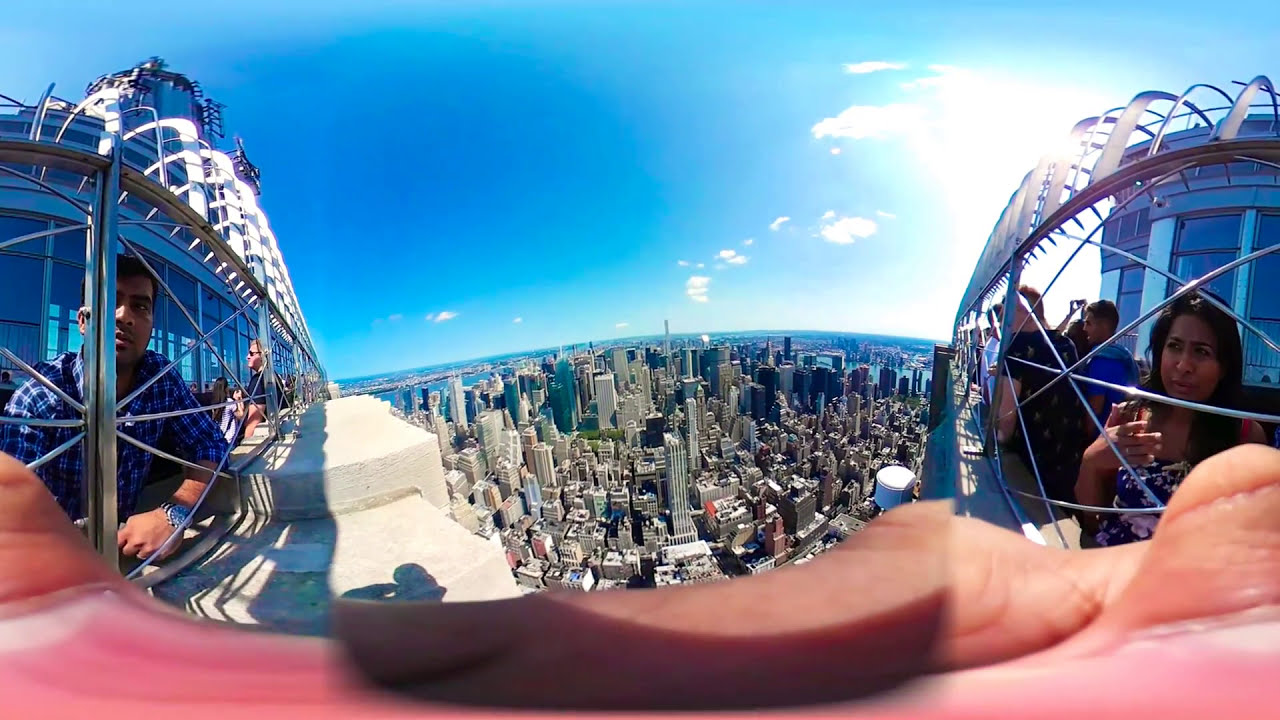The photograph appears to be a 360-degree, slightly warped, bird's-eye view of a bustling city, potentially New York City, with a skyline dominated by tall buildings. The image, captured from a high vantage point, seems a bit blurred at the bottom, likely due to someone's hand or finger obstructing the lens. The sky is a vibrant blue with a few clouds that obscure the Sun on the right side. 

In the foreground, to the left, a South Asian man in a blue plaid shirt, wearing a watch, faces the camera. To the right, a South Asian woman with long black hair in a blue tank top is observed, possibly taking photos with a phone. Behind these individuals, more people, likely tourists, mill about, suggesting a popular sightseeing spot. Both sides of the image display large protective metal barriers with crisscrossing wires, likely for safety. In the background, the cityscape extends into flat land with visible patches of water between some buildings. The structures in the distance, with brown and gray tones and large windows with dark panes, hint at the modern architecture of the location.